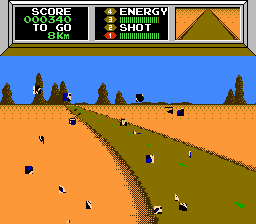The image depicts a vintage, pixelated, 2D video game with graphics reminiscent of 64-bit style. The central focus of the image is a road that begins from the right-hand side and extends towards the middle of the lower right-hand side of the screen. The road is marked by olive green dashes, acting as lane dividers, and is surrounded by an orange playing field. Scattered along the road are blue and black figures that could be interpreted as people or objects, adding to the chaotic scene. At the top of the image, there's a blue sky and a detailed scoreboard featuring the score "000340" and indications such as "8 kilometers to go." The scoreboard also includes sections labeled "energy" and "shot," each represented by green bars. Additionally, the scoreboard has visual representations of the road and various metrics numbered one to four. Brown trees align the screen's top, and an orange wall with blue, black, and white squares lies ahead on the road, suggesting a boundary or obstacle. In the background, mountain peaks or mounds rise, adding depth to the scene. The image conveys a sense of an active, possibly crashed race on a detailed, nostalgia-inducing game screen.